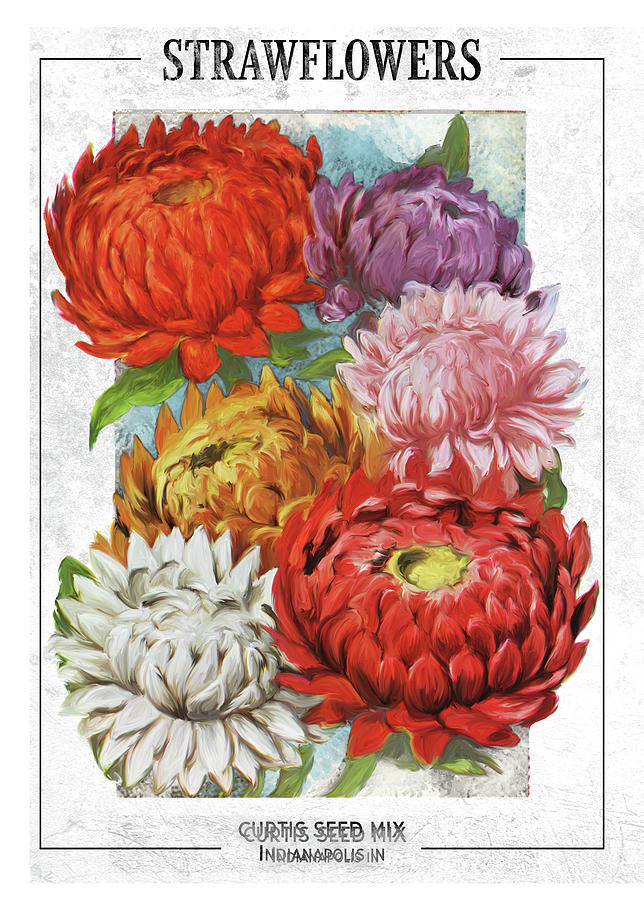This image is a detailed painting of several vibrant straw flowers, depicted in a watercolor style. The composition is bordered by a white frame with a black line running through it. At the top of the image, the title "STRAW FLOWERS" is prominently displayed in all capitalized black font. Along the bottom of the border, the inscription "Curtis Seed Mix, Indianapolis, Indiana" can be seen, suggesting that this image is likely from a seed packet or advertisement for flower seeds.

The flowers themselves are the focal point, capturing the viewer's attention with their large, colorful blooms. The arrangement consists of:

- A red flower with an orange hue at the top left.
- A purple flower at the top right.
- A yellow flower situated in the middle left.
- A pink flower in the middle right.
- A white flower at the bottom left.
- Another red flower with a distinct yellow center at the bottom right.

These vibrant and eye-catching flowers dominate the image, giving a clear and attractive preview of what the "Curtis Seed Mix" promises to grow.